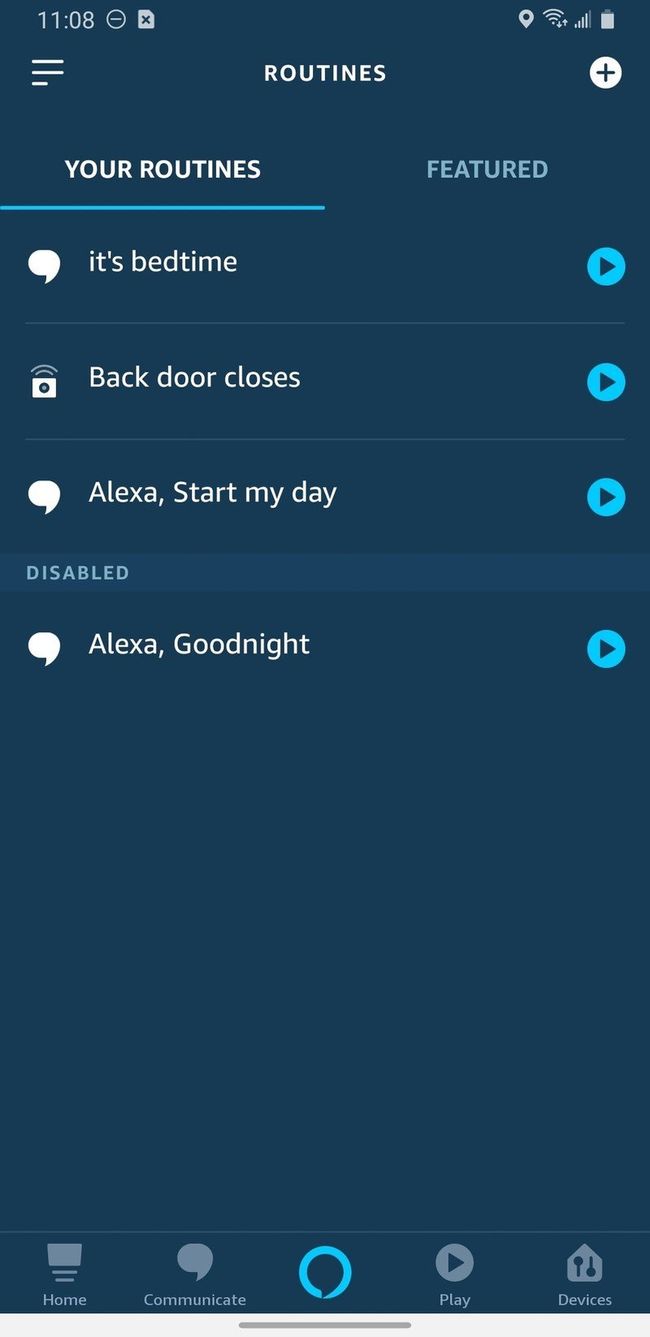The image is a vertically rectangular screenshot from a cell phone, displaying a deep greenish-blue background. At the top center, the word "Routines" is prominently featured, followed by "Your Routines," which is underlined with a blue line, indicating it is the selected tab. In the top right corner, the word "Featured" appears.

Underneath "Your Routines," there is a list of routines labeled "It's Bedtime," "Back Door Closes," and "Alexa, Start My Day." Each routine has a light blue circle on the right side containing a dark blue arrow, signifying a selection tool. Further down, under the heading "Disabled," the routine "Alexa, Midnight" is listed, similarly accompanied by a selection arrow.

At the bottom of the screen, there are navigation options: "Home," "Communicate," "Play," and "Devices." The top of the screen displays the time as 11:08, along with status icons on the right side for location, Wi-Fi, signal strength, and battery life. These icons are situated next to each other, providing relevant information at a glance.